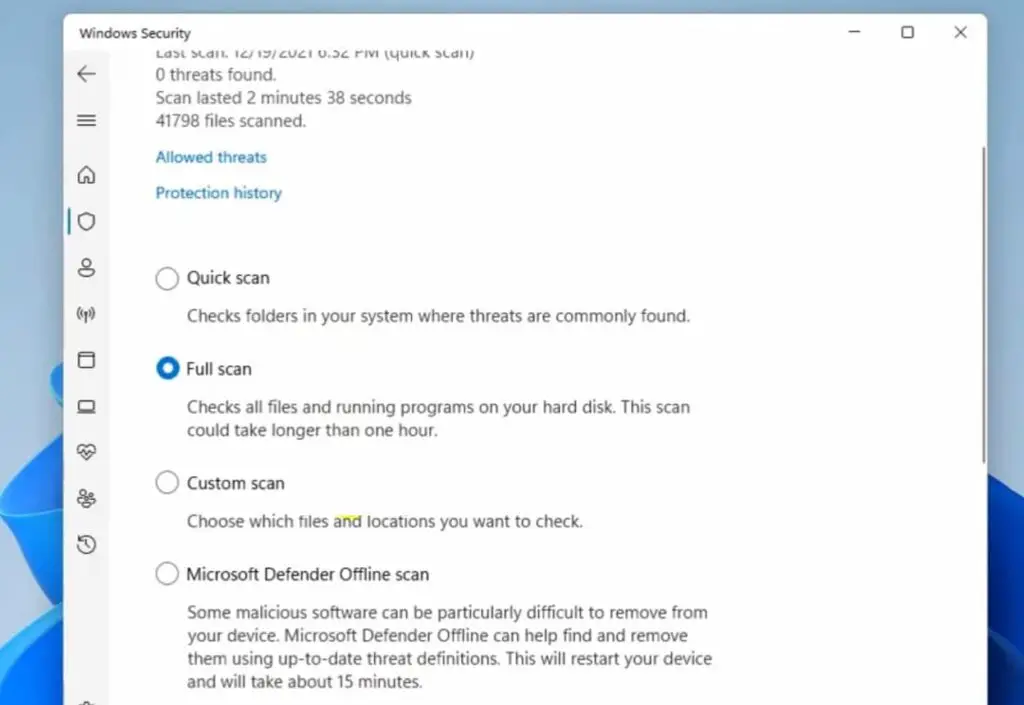Screenshot of an antivirus software interface on a computer screen. The square photo features a blue background with a gradient ribbon effect at the bottom, transitioning from dark blue on the right to light blue on the left. 

In the forefront, a white pop-up window with rounded edges is partially visible. This window is topped by a white header bar displaying the text "Window Security" on the left. 

On the left side of the pop-up, there's a vertical toolbar with icons representing a back arrow, a hamburger menu, a home icon, a shield, a user, a signal, a tab, and a monitor.

The main content of the pop-up provides recent scan details. The text reads:
- "Last scan: 12-19-27"
- "Zero threats found"
- "Scan duration: 2 minutes 38 seconds"
- "41,798 files scanned"

Below this summary, there are two prominent blue buttons labeled "Allow threats" and "Protection history".

Further down, there are four radio button options for different types of scans, each with a header and description:
1. Quick Scan
2. Full Scan - selected with a blue ring around a small white circle, described as "Check all files and running programs on your hard disk. The scan could take longer than one hour."
3. Custom Scan
4. Microsoft Defender Offline Scan